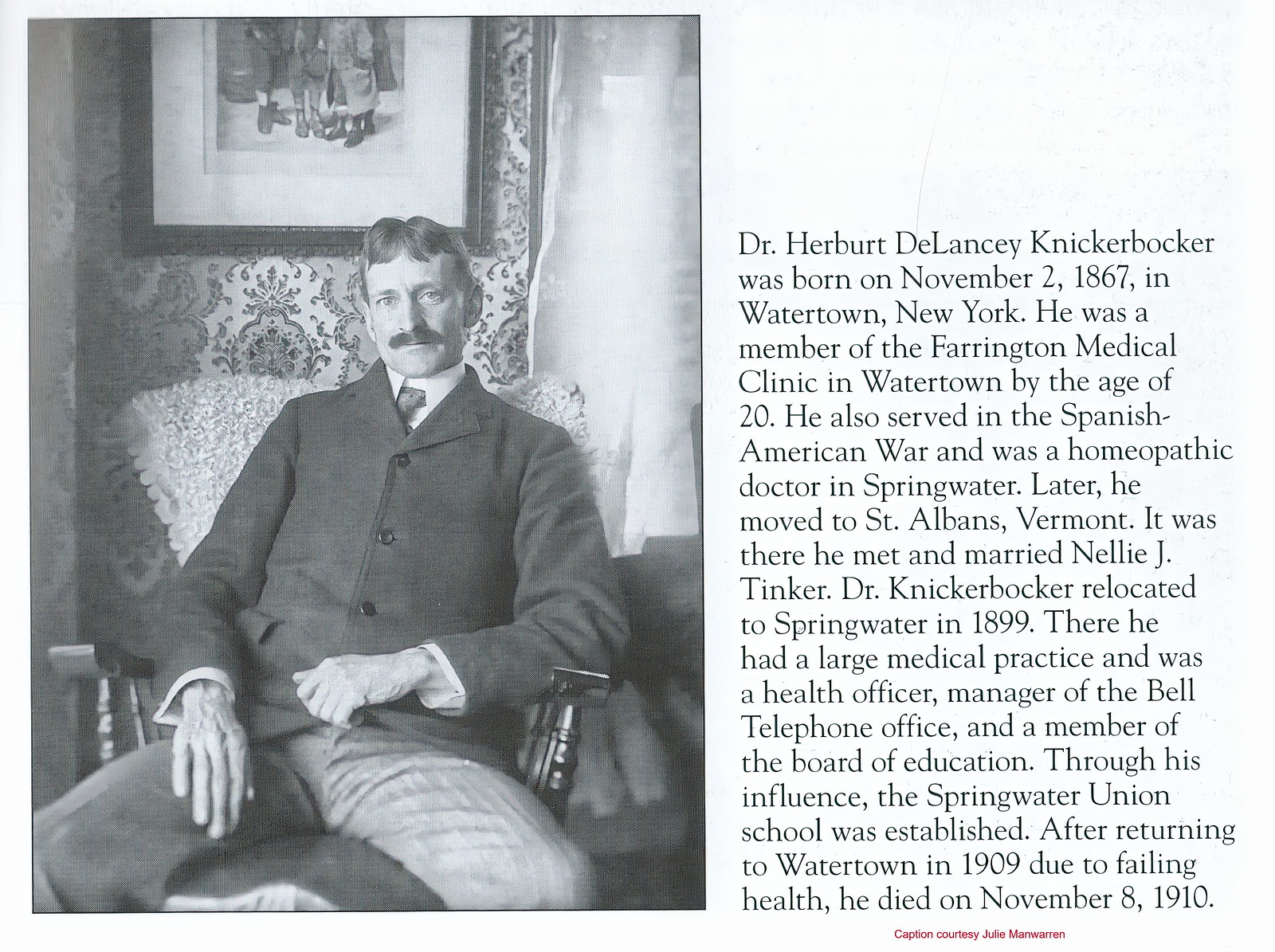This image features an old black-and-white photograph of Dr. Herbert Delancey Knickerbocker, coupled with a lengthy paragraph detailing his life. The photograph, positioned on the left side, captures Dr. Knickerbocker dressed in a dark buttoned-up suit jacket, a white collared shirt, and a tie. With a distinguished moustache, he sits casually in a wooden rocking chair. The room he is in is adorned with a floral patterned wallpaper, and behind him, although partially cropped, is a portrait hanging on the wall.

The text on the right provides a detailed account of Dr. Knickerbocker's life: Born on November 2nd, 1867 in Watertown, New York, he became a member of the Farrington Medical Clinic at the young age of 20. He served in the Spanish-American War and practiced as a homeopathic doctor in Springwater. Dr. Knickerbocker later moved to St. Albans, Vermont, where he met and married Nellie J. Tinker. When he relocated back to Springwater in 1899, he established a significant medical practice, served as the health officer, managed the Bell Telephone Office, and was a member of the Board of Education. His influence was instrumental in founding the Springwater Union School. Due to declining health, he returned to Watertown in 1909 and passed away on November 8th, 1910.